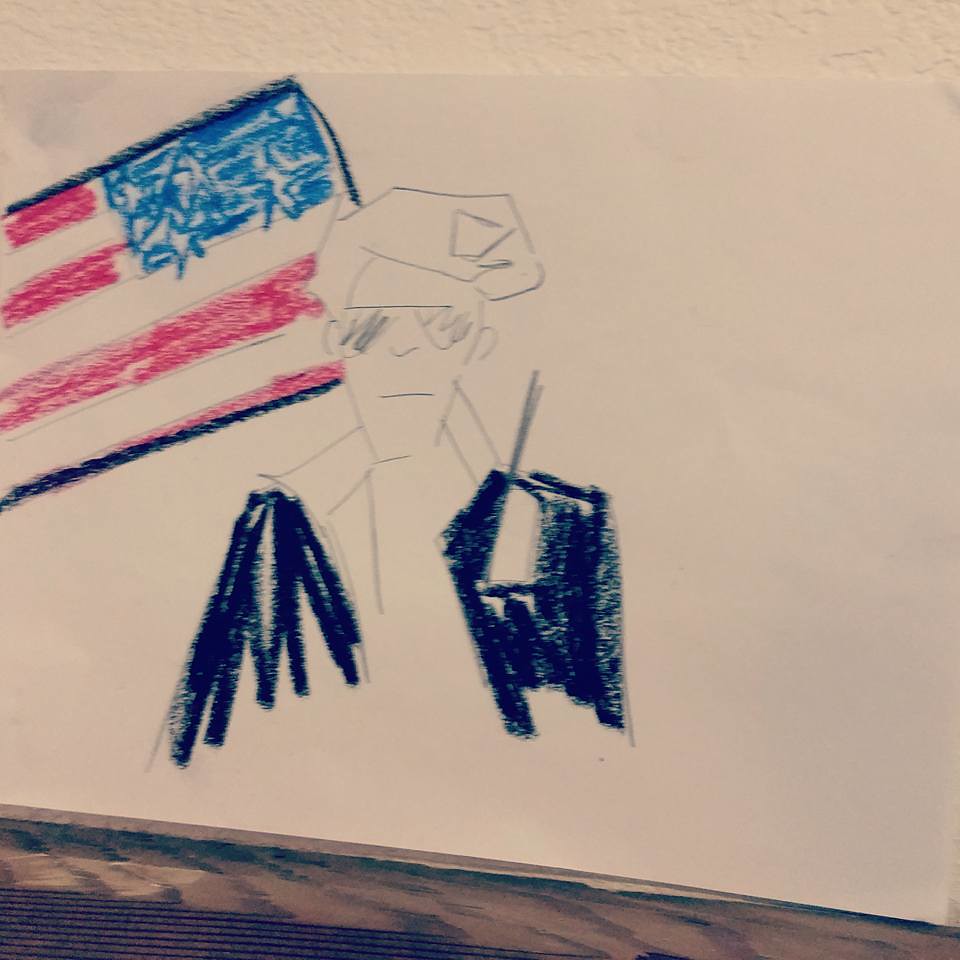In this image, we see a drawing on a piece of white or off-white sketch paper, lying on a wooden desk. The background includes a wooden desk with some lined ridges at the far bottom left, and a white wall at the very top. The drawing combines pencil and crayon work, depicting a man's face and upper body. The man is wearing a hat featuring an insignia in the center, sunglasses, and has a V-shaped nose with a small slit for a mouth. His shoulders are indicated by two lines, and he's partially colored in; his suit jacket is dark blue. There's black crayon scribbling where his hands should be. To the left of the man's image, there's a backward American flag drawn with crayons, with its stars and blue field positioned in the upper right corner. The image captures a distinct, detailed portrayal of a partially colored figure with traditional American symbols.